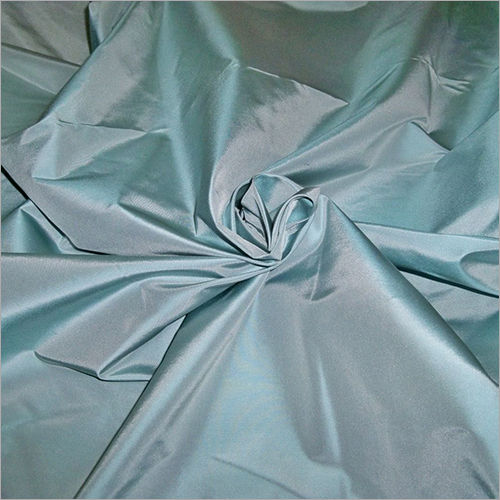The image is a square, low-quality photograph, resembling those taken with older film cameras. It captures a piece of cloth, likely satin or silk, characterized by a sheen and a delightful interplay of colors—primarily a Tiffany blue with hints of silver and light purple where the light reflects. The cloth is splayed out on an unseen surface, possibly a bed, with its central area gathered and twisted into a swirling pattern, giving an impression akin to a flower with spoky ridges radiating outward. The focus of the image is this intricate, wrinkled, and crinkled swirl at the center, emphasized by the harsh, unnatural lighting likely from the camera’s flash. The surrounding material spreads in an irregular, almost chaotic manner, contributing to the overall whimsical and delicate aesthetic of the photograph.